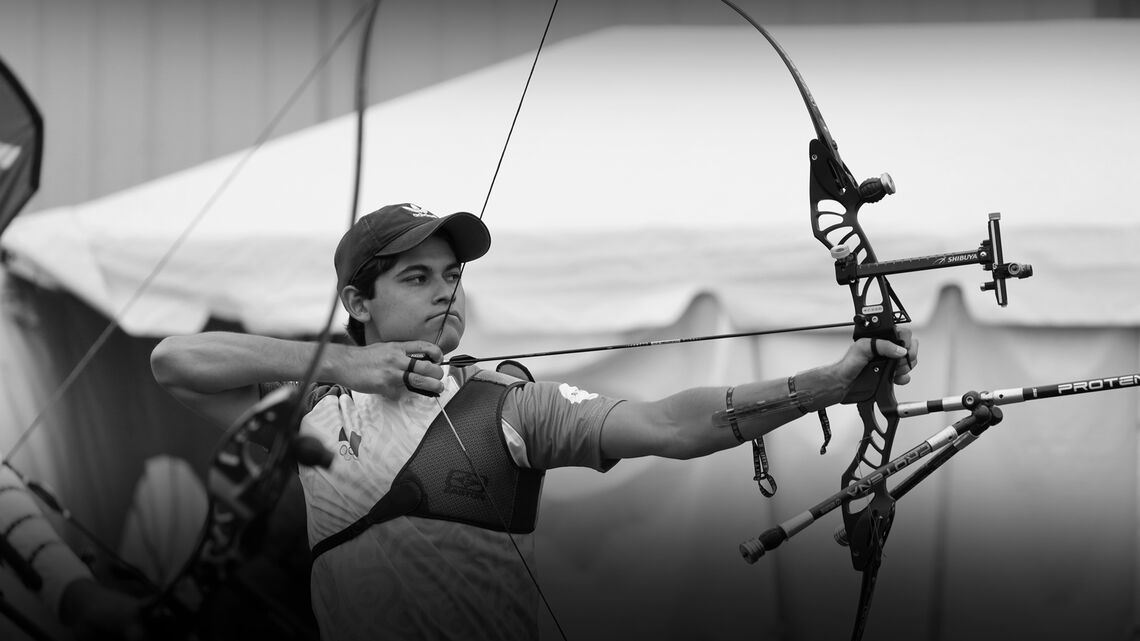This black-and-white outdoor photograph, measuring approximately six inches wide and three inches high, captures a teenage boy engaged in archery. Positioned just left of the center, the boy is seen from the waist up, orienting towards the right side of the image. He wears a baseball cap emblazoned with the Adidas logo and a short-sleeved shirt. Notably, he has a shoulder brace that spans from his left shoulder to the right side of his torso. With a high-tech bow in hand, his left arm extends forward, gripping the front of the bow, while his right arm is bent, drawing the string and arrow back towards his chin, poised to shoot. The bow is sophisticated, featuring numerous attachments around the handle area, likely to aid with precision and stability. A blurred figure is faintly visible on the far left of the image, adding depth to the scene. The background features a white or gray tent, enhancing the monochromatic composition.